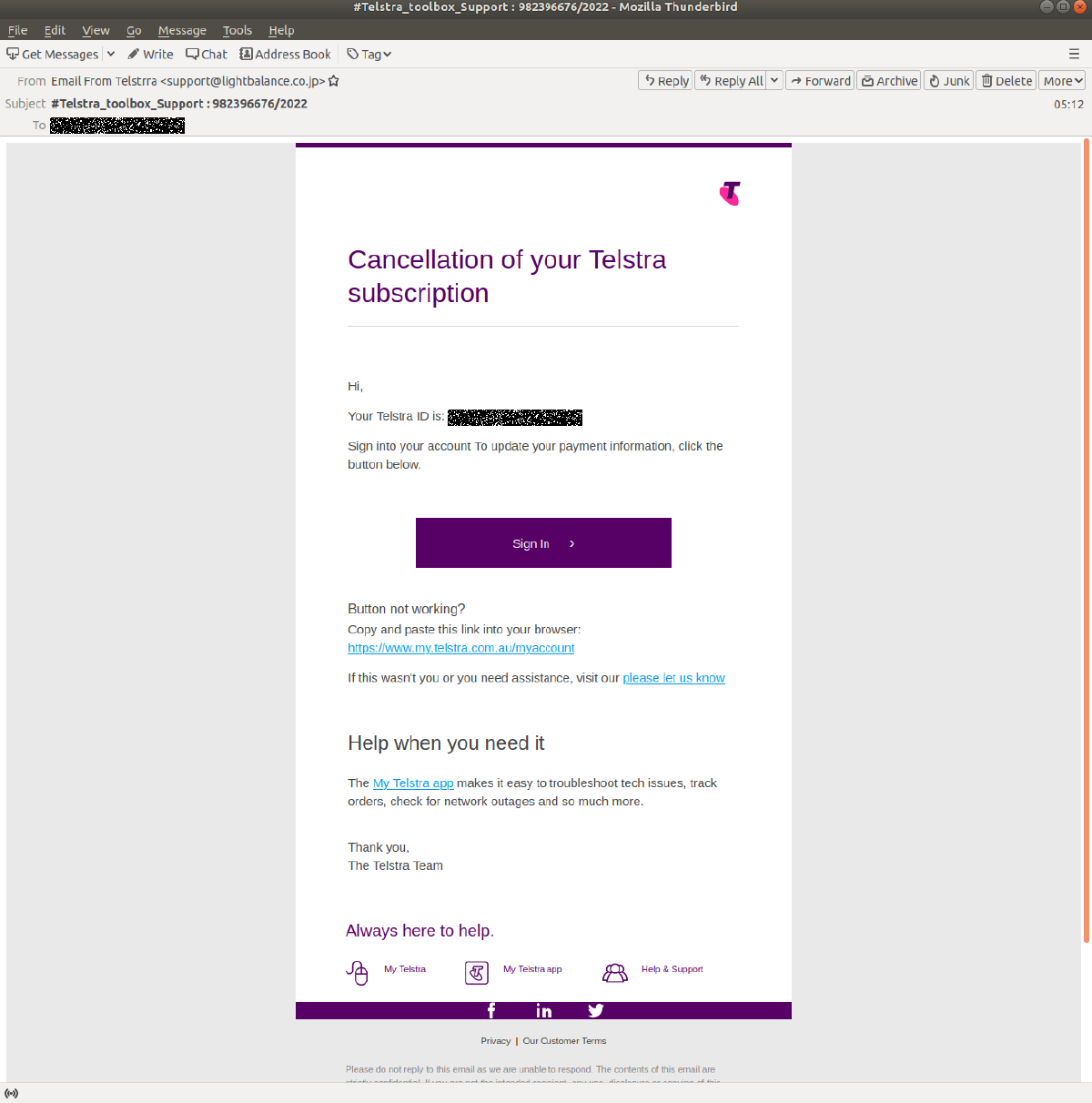Here is a detailed transcription and descriptive caption for the image provided:

---

The image portrays an email message viewed in a page layout format, resembling a typical email client interface, specifically Mozilla Thunderbird. At the top of the interface, there is a gray toolbar that reads "Telstra Toolbox Support 982396676/2022 - Mozilla Thunderbird". This toolbar includes the standard window control buttons: minimize, maximize, and close.

Directly beneath this, there is a secondary menu bar with options labeled “File, Edit, View, Go, Message, Tools, and Help”. Following this, another lighter gray bar features quick-access buttons including “Get Messages, Write, Chat, Address Book, and Tag”.

The message originates from an email address: "Telestra support at lightbalance.co.jp" and is titled "Telstra Toolbox Support 982396676/2022". The recipient's email address in the "To" section is obscured by a black box for privacy. The email client also displays buttons for "Reply, Reply All, Forward, Archive, Junk, Delete," and "More."

The email itself features a white vertical layout with a prominent purple line at the top, along with a purple 'T' logo accompanied by a pink dot background. The email's subject line is "Cancellation of Your Telstra Subscription". The email body starts with a greeting, stating "Hi," followed by a notification that the recipient's Telstra ID (blacked out for privacy) requires an update of payment information. It prompts the recipient to click a purple "Sign In" button to proceed. Below the button, there is an alternative instruction: "Button not working? Copy and paste link in the browser."

For additional support, the email suggests visiting their support page, ending with the message, "If it wasn't you or you need assistance, please visit us now. Help when we need it. The My Telstra app makes it easy to troubleshoot tech issues, track orders, check network outages, and so much more."

The email concludes with a thank you from the Telstra team, emphasizing their commitment to support: "Thank you, the Telstra team, always here to help." Finally, it mentions the My Telstra app and provides links for further help and support, highlighted by Facebook, LinkedIn, and Twitter icons at the bottom.

---